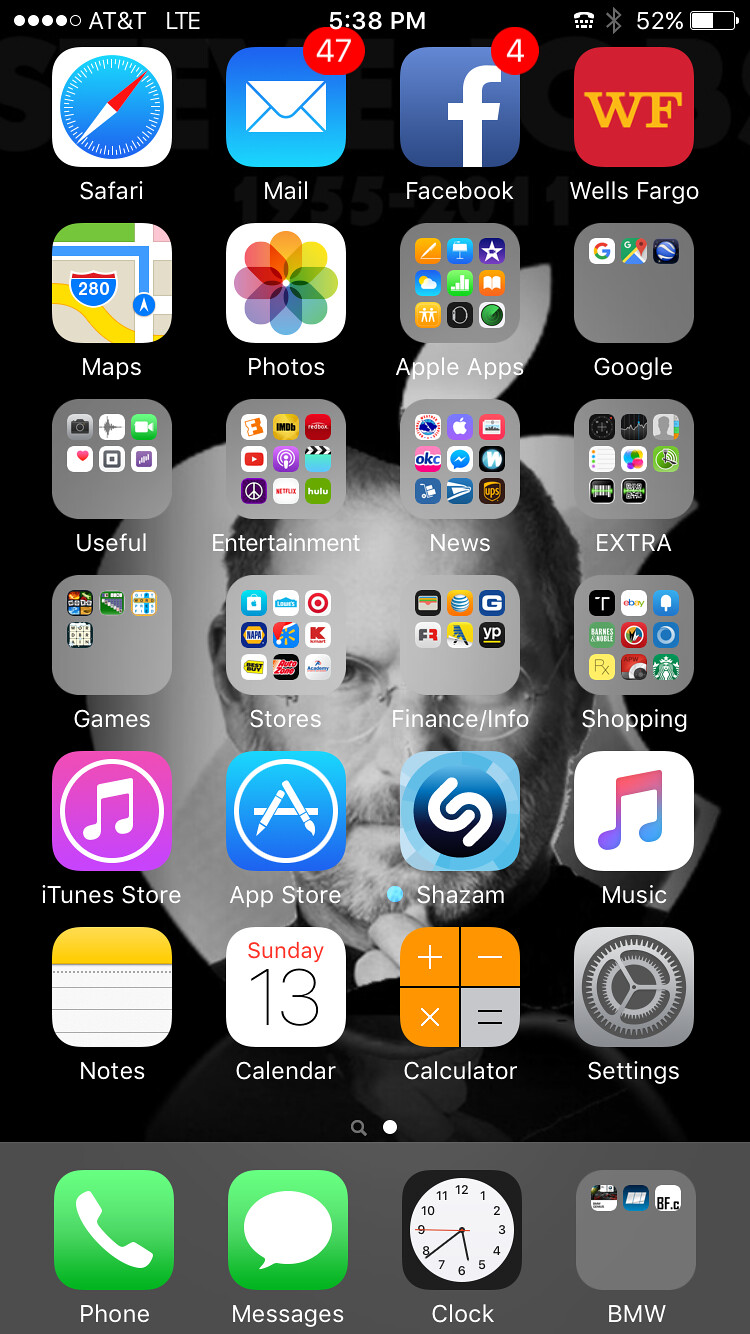A detailed image of a smartphone screen is depicted. The top left corner displays the network status with four out of five bars lit, indicating strong AT&T LTE service. The time is shown as 5:38 p.m., and the battery meter indicates a 52% charge, with the battery icon split equally into black and white. The wallpaper features a striking, black-and-white photograph of a man who resembles Steve Jobs. He has wireframe glasses, a salt-and-pepper mustache and beard, thinning hair, and is posed with his hand on his chin, suggesting deep contemplation.

In the foreground, there are six rows of app icons, each row containing four apps. The top row showcases Safari, Mail (with 47 notifications denoted by a red circle), Facebook (with 4 notifications in a red circle), and Wells Fargo. Other recognizable icons include Maps, Photos, Google, Games, iTunes, and the App Store, among others. The bottom gray bar features a phone app represented by a white phone icon in a green square, a messaging app with a green message bubble icon, a clock icon, and a BMW app. The palette of the screen contains various colors such as black, white, red, blue, yellow, and green.